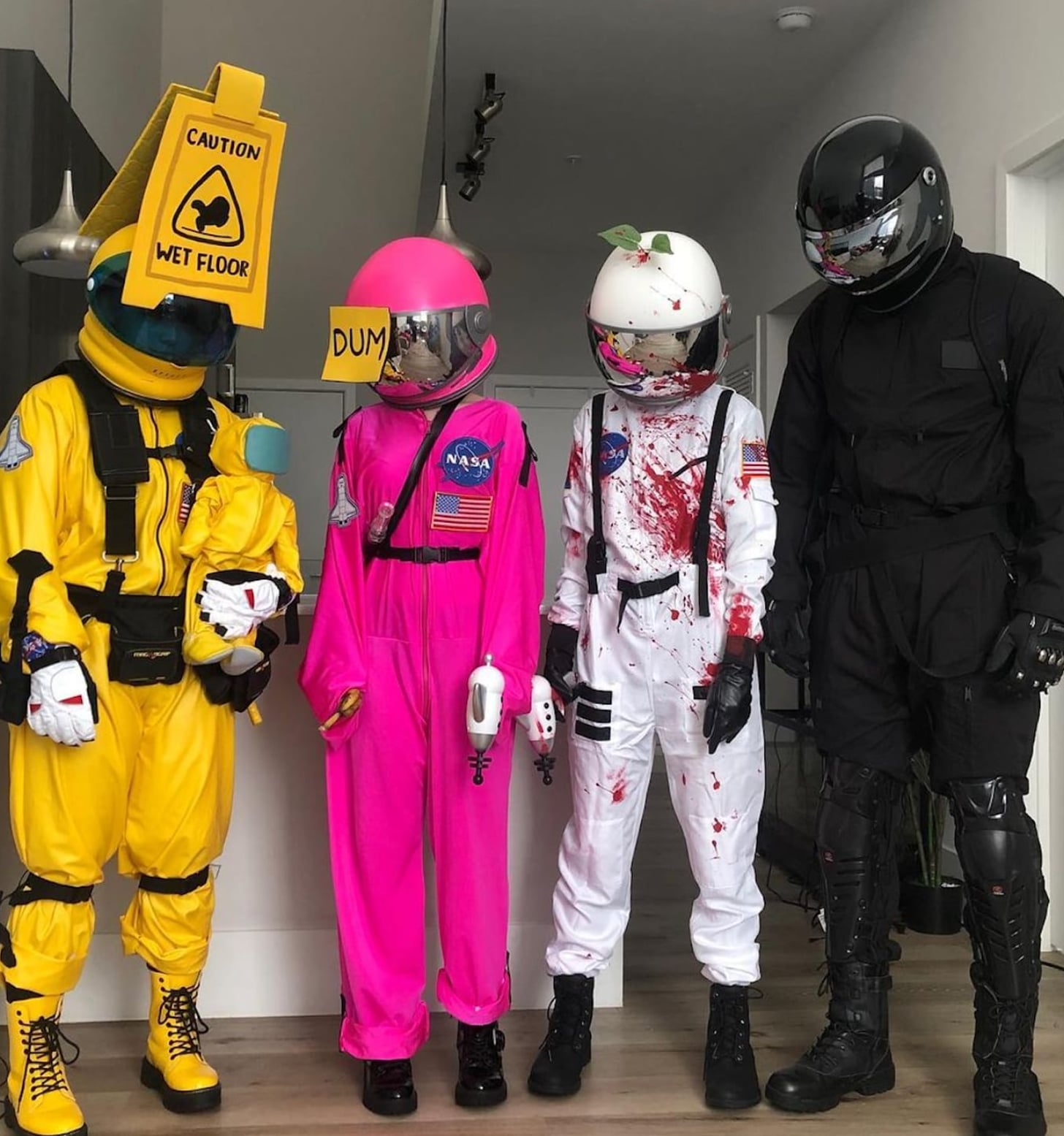The image showcases a detailed and imaginative Among Us-themed cosplay or art installation featuring four astronaut suits. Each suit appears to be customized to reflect different personalities or roles from the game. The figures are posed in a vertical alignment, with three of similar height and one notably taller figure on the far right.

Starting from the left:
1. The first suit is a distinctive yellow astronaut outfit adorned with black accents. It features a yellow "Caution: Wet Floor" sign affixed to the helmet. The figure is holding a smaller, yellow astronaut doll in its left arm, adding a whimsical touch.
2. Next, a pink astronaut suit stands out with "NASA" and the United States flag displayed prominently. This figure has a post-it note labeled "DUM" stuck on its pink helmet. Both the pink and white suit-wearers hold space-themed "ray guns."
3. The third figure dons a white astronaut suit, complete with a white helmet. Notable for a dramatic element, this suit is splattered with faux blood, creating a striking visual contrast. Small, decorative leaves are placed atop the helmet, enhancing the eerie yet artistic design.
4. The final suit, towering over the others, is entirely black. This figure wears a black helmet reminiscent of a motorcycle helmet, complete with armored shin guards and knee pads, giving it a more solid and formidable appearance.

All figures are equipped with gloves and sturdy black boots, contributing to the overall uniformity and cohesiveness of the display. This inventive setup appears to be a creative representation of characters from the popular video game Among Us.